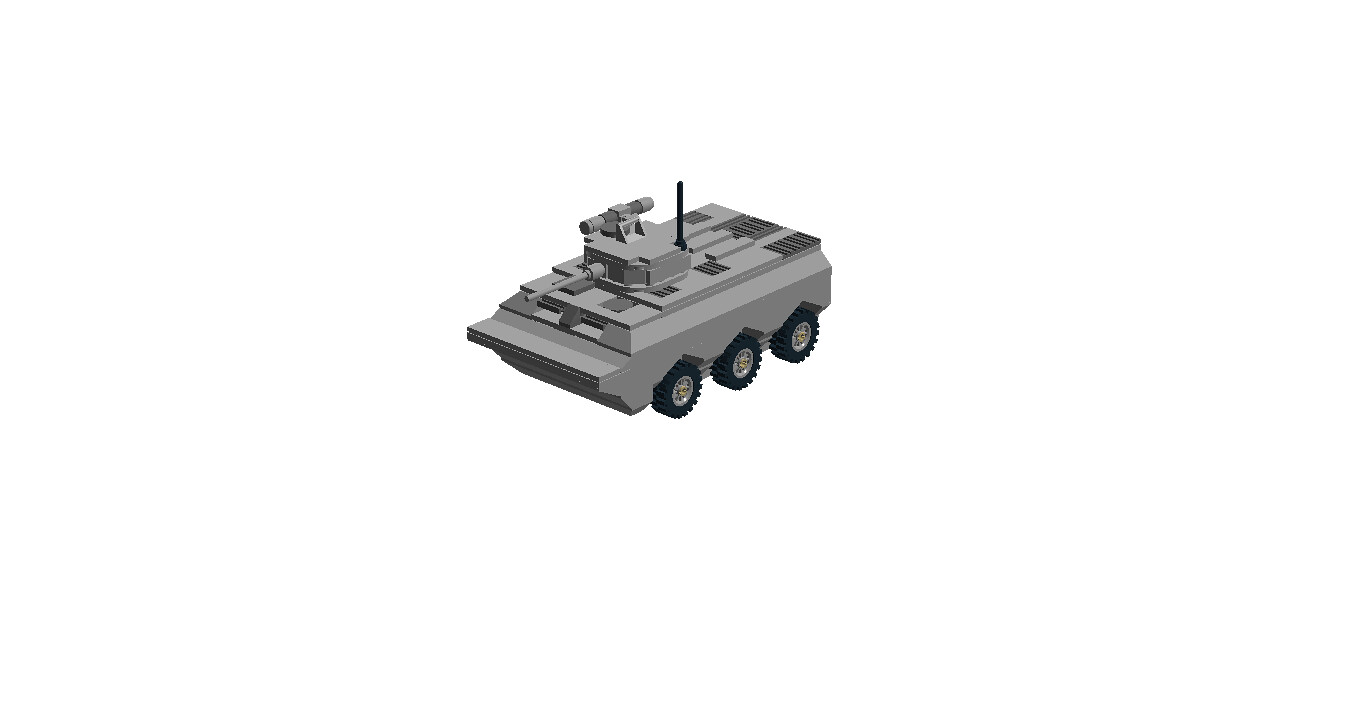This image displays a computer-generated, cartoon-like representation of a light gray tank. Rendered in a CAD program, the tank is positioned diagonally, with its front facing the lower left-hand corner. Three prominent black wheels are visible on the side closest to the viewer, suggesting an equal number on the opposite side. The tank's moderately sized turret houses a short, unimpressive cannon that does not extend past the vehicle's front. An antenna protrudes from the top of the tank, giving it a multi-leveled appearance. The background is a stark white, emphasizing the tank's gray hue and minimalist design. The overall aesthetic is reminiscent of a tank emoji, simple yet detailed enough to convey the essential features of the vehicle.